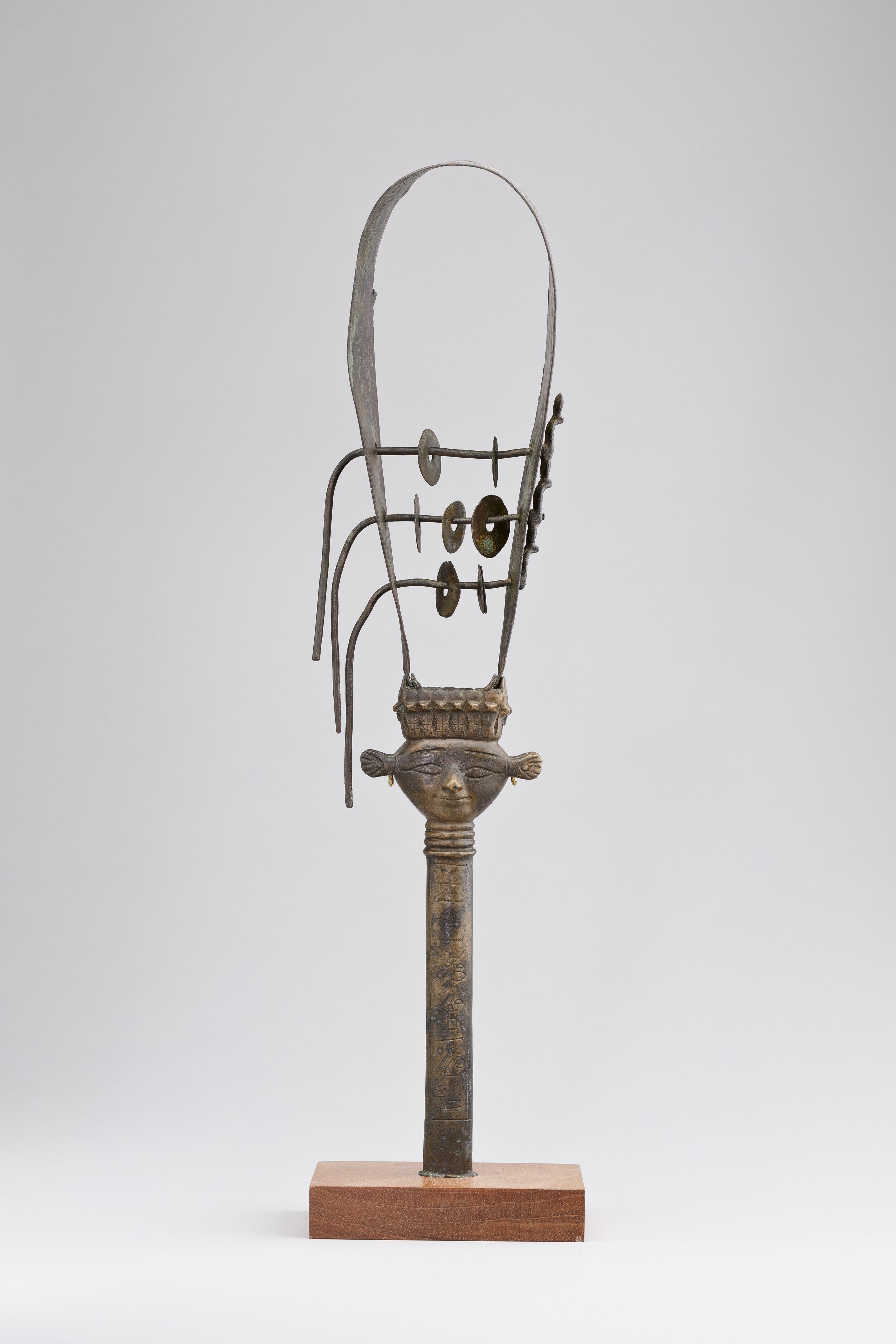This image showcases a bronze-like metal sculpture affixed to a small wooden block, standing against a stark white background that encompasses both the surface and backdrop. The sculpture, which has an ancient, perhaps Egyptian or African aesthetic, features a thin, roughly foot-long metal pole adorned with intricate markings. Atop this pole is a metal face with long, drawn-out eyes and prominent ears that appear to have earrings dangling from them. Crowning the head is a rectangular ornamentation resembling a basket or a hat, from which a tall U-shaped metal arc extends upward, nearly as tall as the sculpture itself. This arc has horizontal metal wires piercing through it, from which multiple rings or washers hang, creating an effect reminiscent of beads or parts of an abacus. The interplay of these elements, set against the pure backdrop, evokes the impression of an artifact from a museum's carefully curated collection.